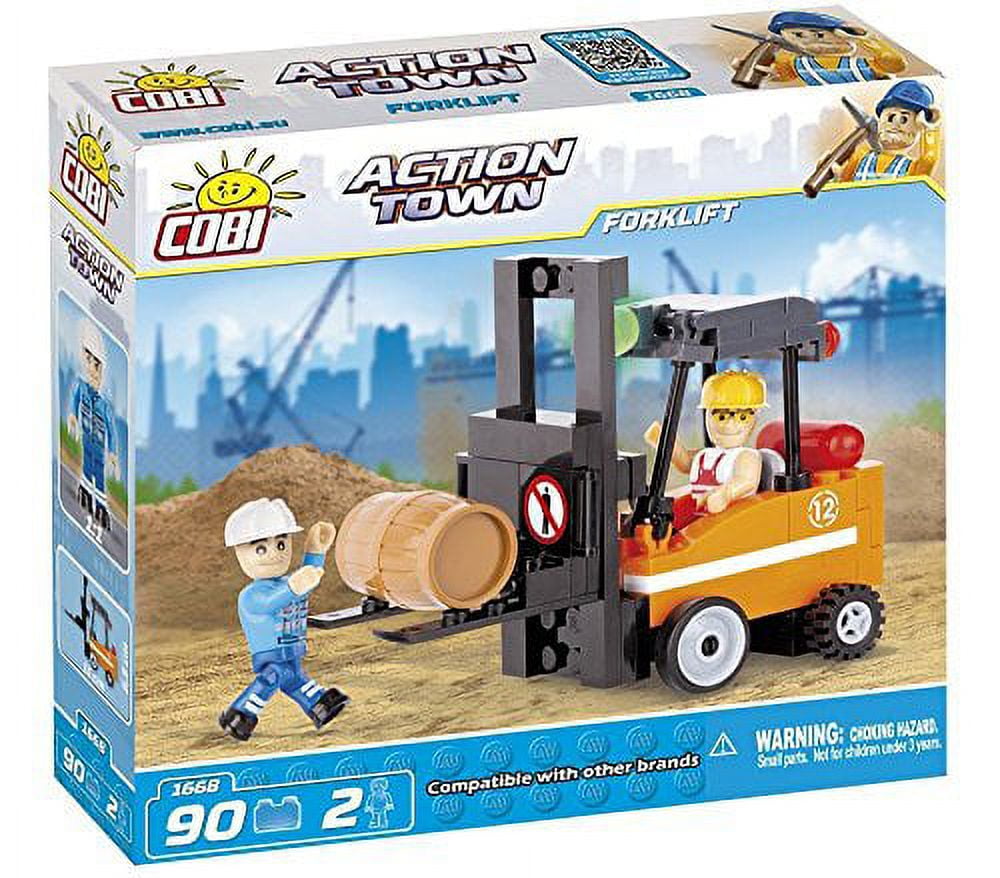The image displays a detailed photograph of a product packaging reminiscent of Lego sets, showcasing a toy forklift scene. The focal point is an orange forklift with black panels and a red seat. The forklift is operated by a figure dressed in red and white overalls and a yellow hard hat. Adjacent to the forklift stands another figure in a light blue shirt and dark blue pants, donning a white hard hat, efficiently loading a brown barrel onto the forklift. 

The box's background illustrates a vibrant construction site with cranes, buildings, bridges, and a water body, adding depth and context to the scene. Prominently at the top of the package, "Forklift" is written in white letters, with "Action Town" slightly lower to the right and "COBI" in white with a red outline to the left, along with a cheerful yellow sun logo featuring the word "Kobe." 

Further details on the packaging indicate the set includes 90 pieces, denoted by a "90" next to a block piece, and two figures, indicated by a "2" next to an image of a figure. Labels on the lower part of the box state the contents are compatible with other brands and include a warning about potential choking hazards.